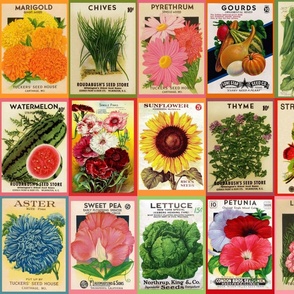The image displays a vibrant 4 by 3 grid of various seed packets, meticulously arranged to form a cohesive compilation of flowers and herbs. The first row features marigolds in vibrant orange and yellow hues in the top left corner, followed by chives, then pyrethrum with pink and white blooms, and ending with gourds. The second row begins with watermelon, then proceeds to red, white, and pink flowers, sunflowers, thyme, and finally, strawberries. The last row showcases aster flowers in blue, sweet peas in pink, green lettuce, and concludes with petunias in shades of white, burgundy, and dark pink. Each seed packet is vividly illustrated, making this collection an eye-catching and desirable assortment for any gardening enthusiast.